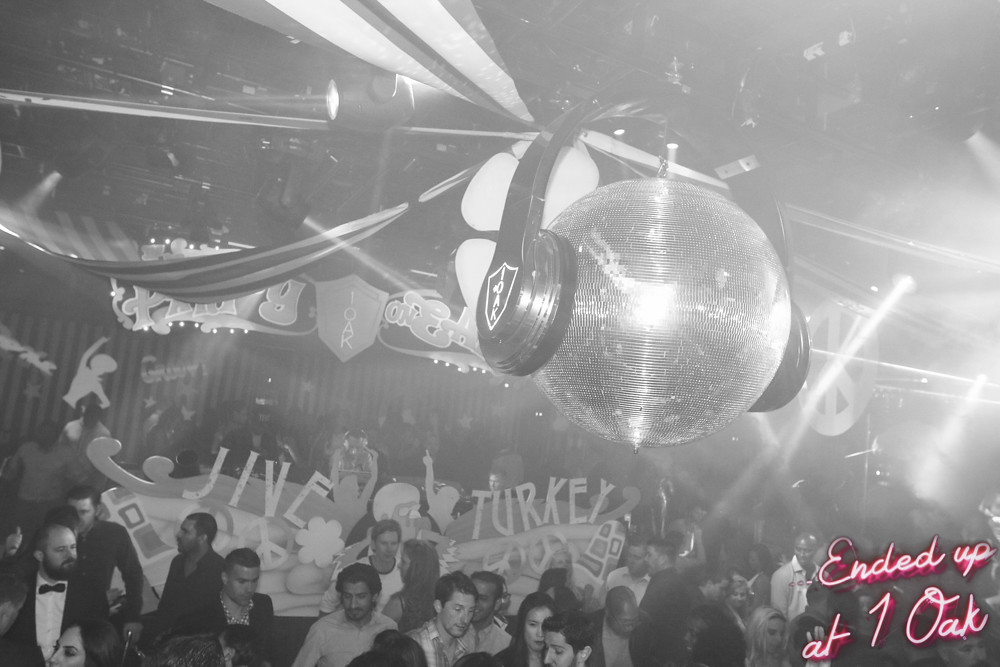In this black and white image of a nightclub scene at One Oak, a prominent disco ball adorned with a large headset dangles slightly off-center to the right from the ceiling, casting a nostalgic shimmer over the space. Surrounding the disco ball, decorative streamers and signs add to the festive atmosphere, while faint, smoky haze contributes to the hazy ambiance of the room. Below the disco ball, the dance floor teems with the heads of partygoers, either dancing or mingling beneath the dim lights. Text reading "Jive Turkey" appears in the background, set against the smoky backdrop. In the bottom right corner, a neon-like sign in red and white proclaims "Ended at One Oak," adding a splash of brightness to the monochrome setting.